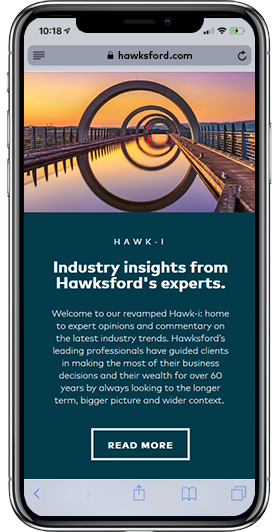This is a detailed screenshot of a smartphone displaying a web page. At the top of the screen, the time reads 10:18 AM, with two bars of cellular coverage, full Wi-Fi signal, and a battery at approximately 50% life. The search bar at the top includes a black padlock icon, indicating a secure connection, and shows the URL "hawksford.com."

The central part of the screen features a captivating photograph of a series of elegantly curved bridges spanning a narrow body of water. The curves create a mesmerizing optical illusion as they reflect in the calm water, forming what appears to be solid, concentric circles. The backdrop is a stunning gray and orange sunset, adding a serene ambiance to the image.

Under the photograph, the text reads: "hawk-1. Industry insights from Hawksford's experts. Welcome to our revamped Hawk-I, home to expert opinions and commentary on the latest industry trends. Hawksford's leading professionals have guided clients in making the most of their business decisions and their wealth for over 60 years by always looking to the longer term, bigger picture and wider context."

Below this text is a white-bordered rectangle with the words "Read More" in white lettering, inviting further exploration of the content. The image is vertically oriented and contains no human subjects.